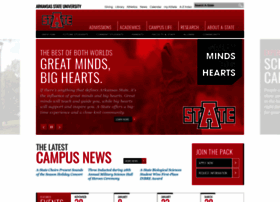This image displays the official website of Arkansas State University. In the upper left-hand corner, the university's name is prominently featured. A search bar is located in the upper right-hand corner, though the text in between is too small to discern. The website is bordered in red, featuring the state logo, in which the letter "A" is significantly larger than the other letters in "STATE." The primary navigation bar includes sections labeled "Admissions," "Academics," "Campus Life," "Research," and "About State."

Center frame showcases an image of three young women dressed casually in jeans and hoodies, walking along a path flanked by greenery. Overlaying this image is the text: "Welcome to Arkansas State. Find your place in the pack." Below this section, there is an area with a white background that highlights "The Latest Campus News." Adjacent is a red background section labeled "Join the Pack," featuring black entry points for applications, though one of these points is indistinguishable due to small text size.